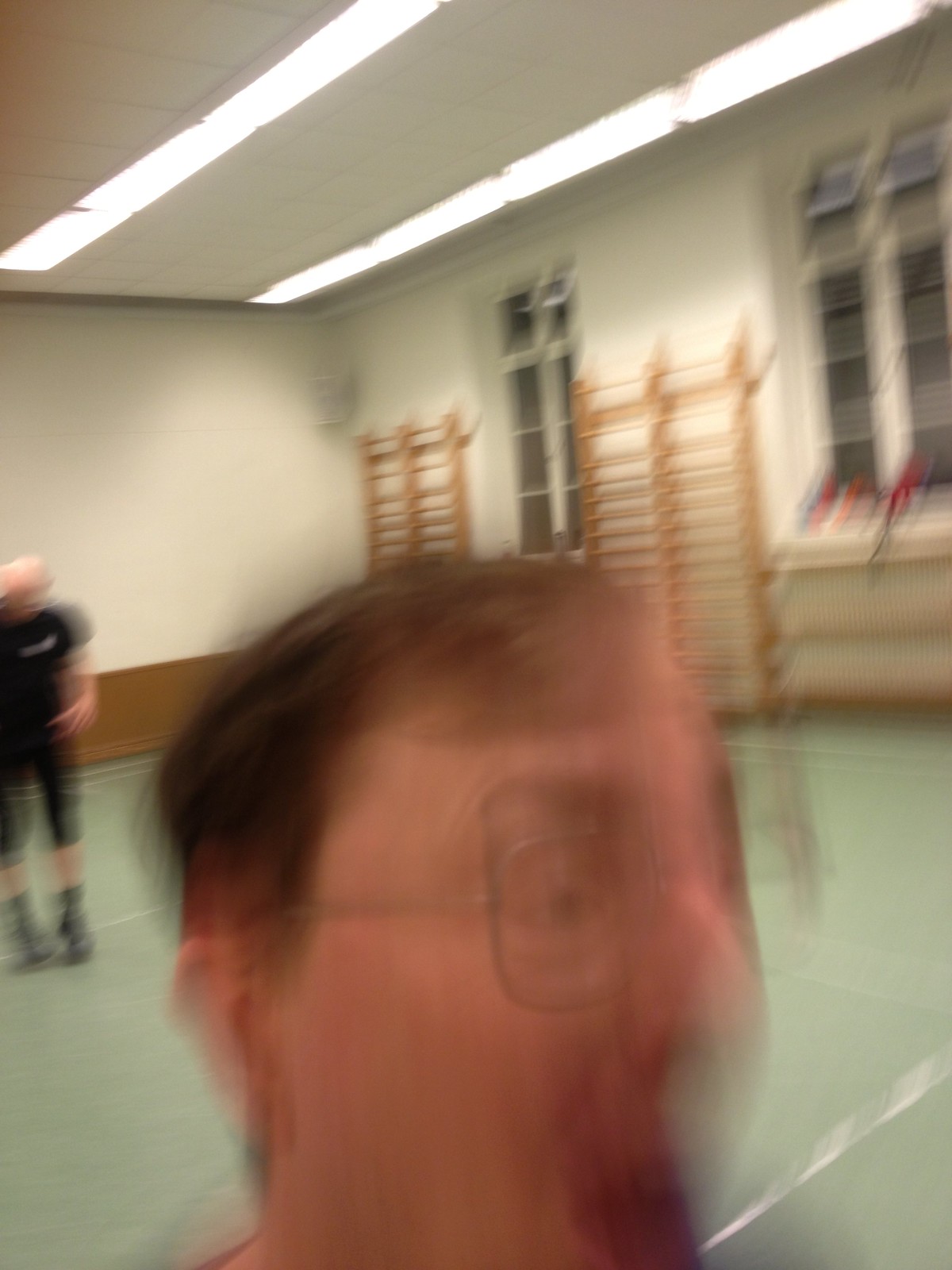In this blurry image, a surprised or shouting white man with short brown hair and large silver-rimmed glasses stands in what appears to be a PE room or sports hall. The man is positioned on a green court marked with white lines around the perimeter and through the middle. In the background, a bald man dressed in a black t-shirt, black shorts, and black trainers stands some distance away, observing the scene. The walls of the room are light-colored, possibly white or off-white, adorned with wooden climbing frames or bars. Additionally, two large multi-paned windows are visible, either with closed panes or showing darkness outside. The overall atmosphere suggests an indoor sports facility, with elements typical of a school gym or recreational space.